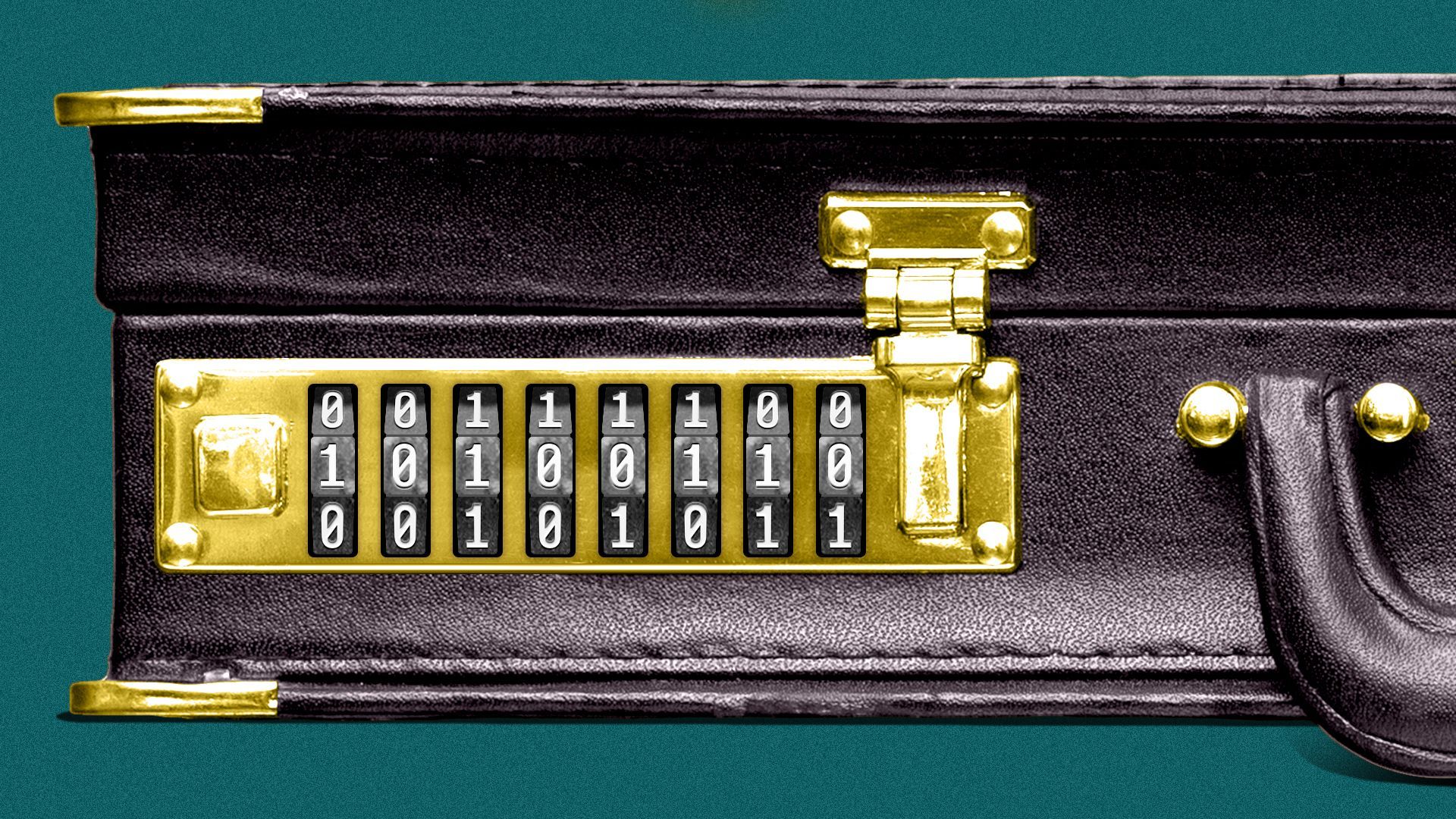This detailed image showcases a sophisticated black leather briefcase set against a teal background. The briefcase, made of high-quality leather with visible stitching, features a golden combination lock in the center of its front cover. This lock has eight small black dials with white numbers, primarily zeros and ones, set to the sequence 10100110. The briefcase is partially seen, with the left side of the handle just visible on the right edge of the image, and the base of the handle affixed with golden ball fasteners. The corners of both the lid and the bottom of the briefcase are reinforced with gold or brass metal to resist wear. Additionally, the composition is zoomed in on the left half, focusing on the intricate details of the locking mechanism, which includes a small lever and a large rectangular plate. The briefcase sits on its side, showcasing its elegant and durable design against the contrasting teal background.